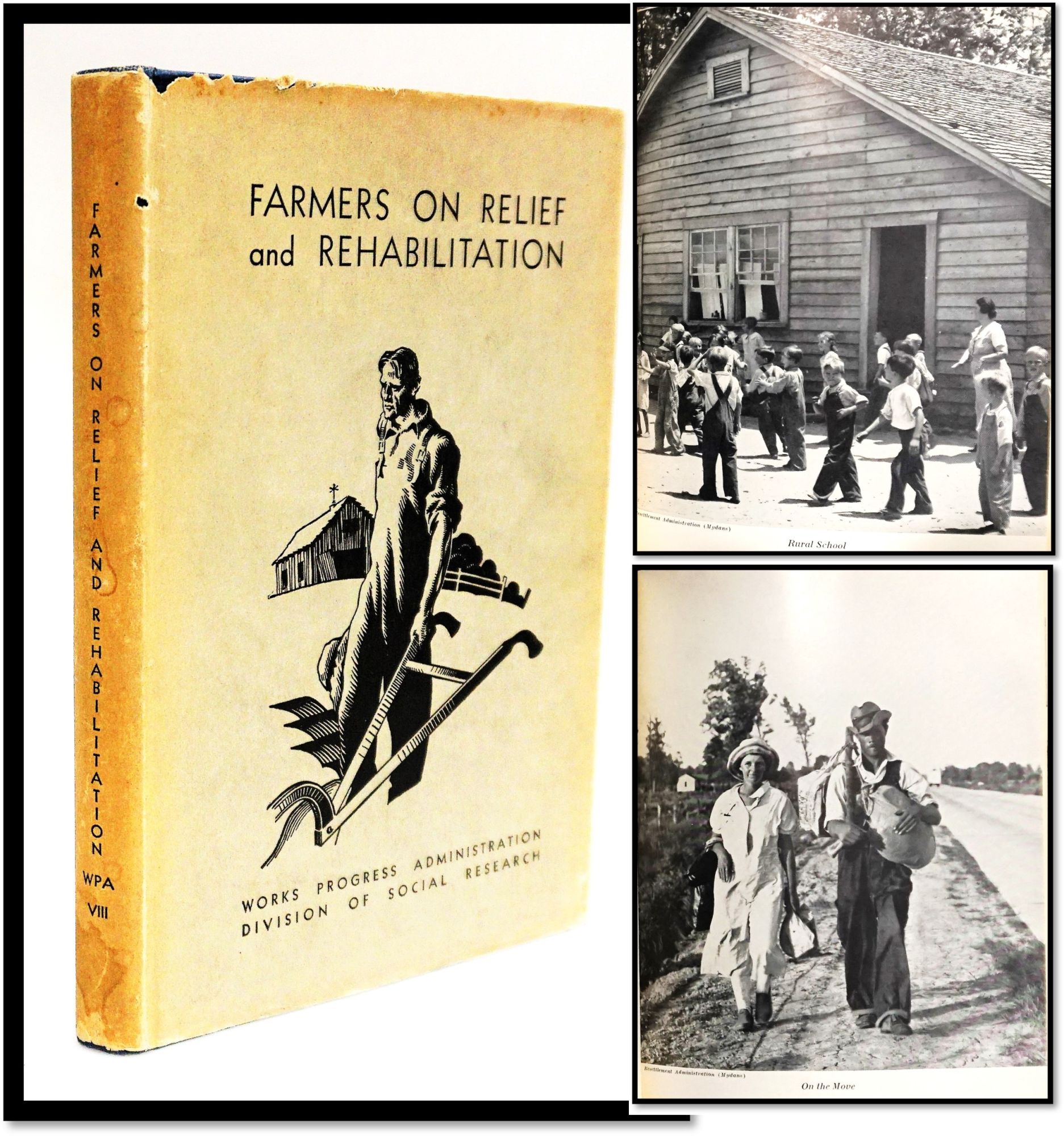This image features a framed composition with three distinct sections capturing the essence of the 1930s-era agricultural life and programs aimed at farmer rehabilitation. The primary focus is a book standing on its lower edge, titled "Farmers on Relief and Rehabilitation," published by the Works Progress Administration (WPA) in 1931. The book's cover, now yellowed with age, prominently displays a stark black and white illustration of a sad-looking farmer holding a tilling instrument. He is depicted standing before a farmhouse, symbolizing the struggles and the eventual aid provided by various New Deal initiatives post the Great Depression.

To the right of the book are two vertically-oriented black and white photographs from the same era. The upper photograph depicts a group of around 15 to 20 children and a teacher gathered in front of a simple wooden schoolhouse with a shingle roof, suggesting rural education during this period of rehabilitative efforts. The lower photograph shows an African-American farmer couple walking down a road, the woman in an ankle-length white frock with a bonnet and the man in overalls and a tilted fedora, each carrying bags. The imagery collectively highlights the socioeconomic backdrop and the focus of the WPA's relief and rehabilitation programs for farmers and their families during the 1930s.